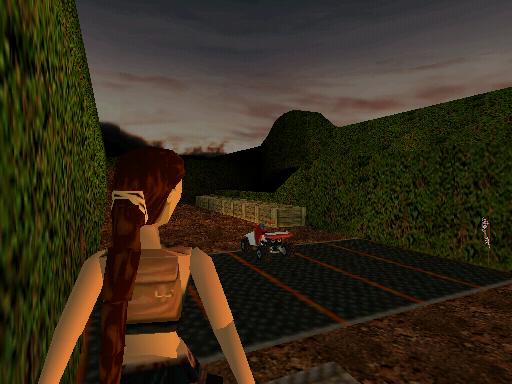A detailed descriptive caption could be: 

"In this animated scene, a woman with long, flowing red hair that cascades down to below her waist stands with her back to the viewer. She is outdoors, surrounded by tall, dense green shrubs that rise above her head, creating a natural wall of foliage. The setting exudes a rustic charm, enhanced by the presence of a small utility vehicle, similar to a lawnmower but without blades, suggesting a farm or open land environment. Scattered around are wooden crates, possibly used for transporting materials. The ground is a rough, unpaved brown earth, adding to the authenticity of the rural atmosphere. The sky hints at an approaching sunset, casting a warm glow over the scene."